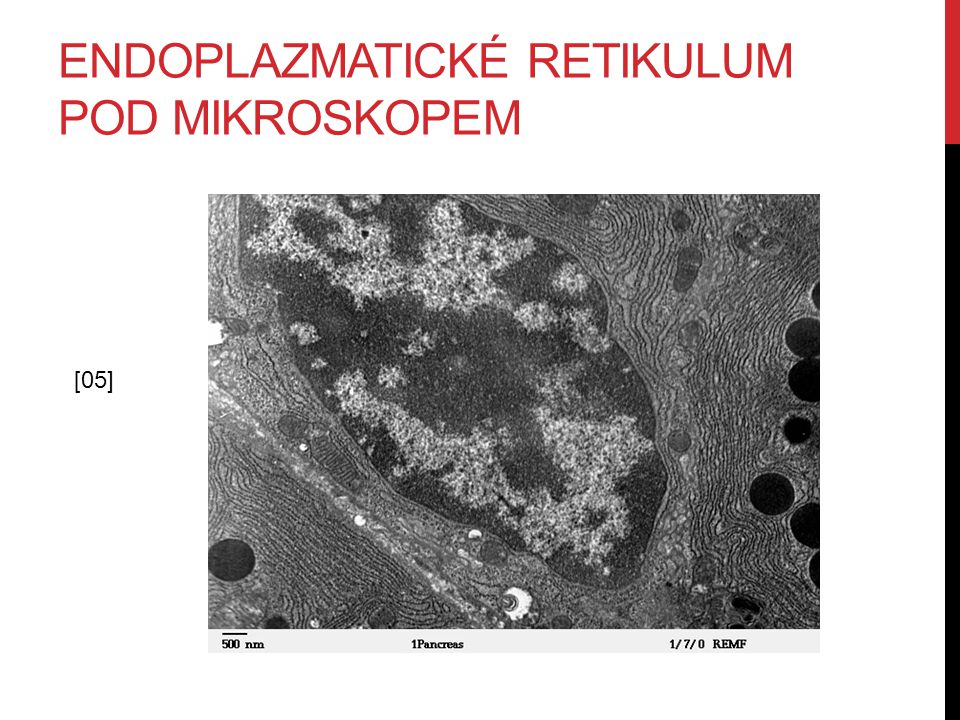The detailed image appears to be a highly zoomed-in, low-quality micrograph, possibly taken from a scientific presentation or medical context. The photograph, labeled "pancreas" at the bottom, predominantly features red, white, black, and various shades of gray, showcasing the intricate structures of cells, likely from the pancreas. At the top of the image, in red text and a different language, it reads "endoplasmatic reticulum pod microscopum." Additional text includes the number "500 nm" at the bottom left and "1/7/0 REMF" at the far right. The image and text are somewhat off-center to the right, emphasizing the detailed cellular formations within the pancreas.